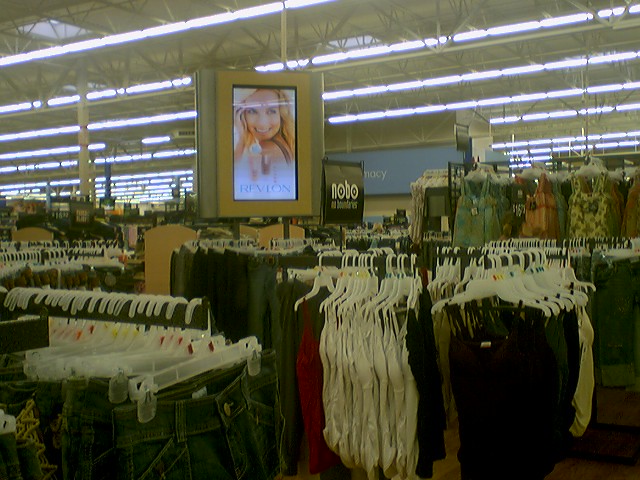This low-quality, old-style landscape photo captures the interior of a bustling department store, likely a Walmart or similar big-box retailer. The image focuses on the women's clothing section, prominently featuring various racks filled with denim jeans, jean shorts with clear hangers, bodysuits, and camisoles. Toward the bottom left, there's a rack of jean shorts, while the middle showcases bodysuits and summer dresses with blue, pink, and yellow flowery designs. To the far right, more dresses are visible. The store is brightly lit with large horizontal fluorescent lights neatly aligned across the ceiling, which includes structural support beams. In the center of the image hangs a prominent illuminated Revlon advertisement featuring a smiling woman with blonde hair, accompanied by the brand name in bold white text. A blue pharmacy sign partially reading "MACY" is seen at the back, suggesting it might be the edge of a sign for the pharmacy area. Additionally, there’s a black square sign with white letters that says "NOBO" visible in the background, indicating the juniors' clothing brand "No Boundaries." The image is rich in detail and provides a nostalgic glimpse into a vibrant retail environment.